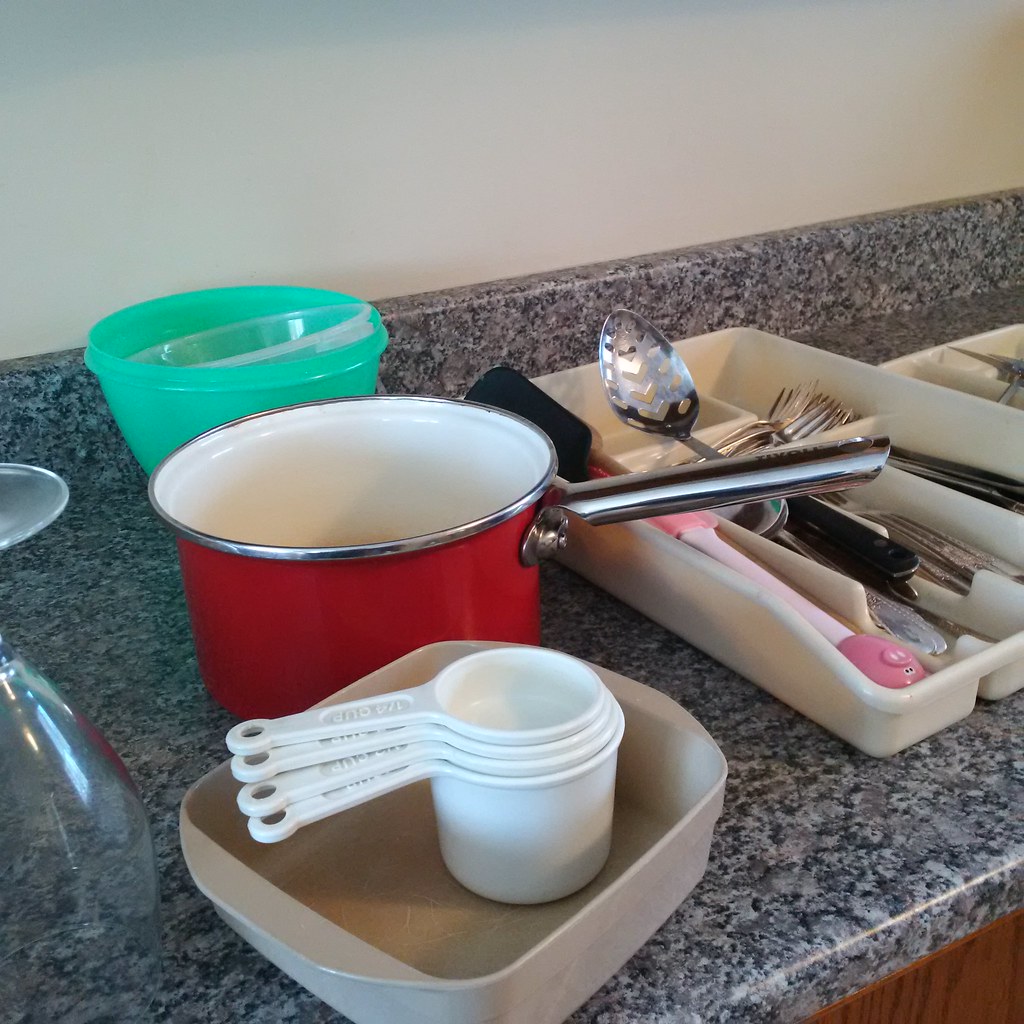On a marbled gray kitchen countertop, various objects are neatly arranged. To the left, an upside-down fluted glass is partially visible, its silhouette cut off by the frame. Centrally positioned is a square, translucent plastic baking pan, containing a set of white stacked measuring cups. Directly behind the pan sits a vibrant red saucepan with a white interior, its silver handle extending to the right. Further back, a seafoam green Tupperware bowl adds a pop of soft color. To the right, an off-white plastic utensil tray holds an assortment of utensils: forks, a slotted spoon, and a pink rubber spatula with a white handle. Just beyond this tray, the corner of another white plastic utensil tray is faintly visible.